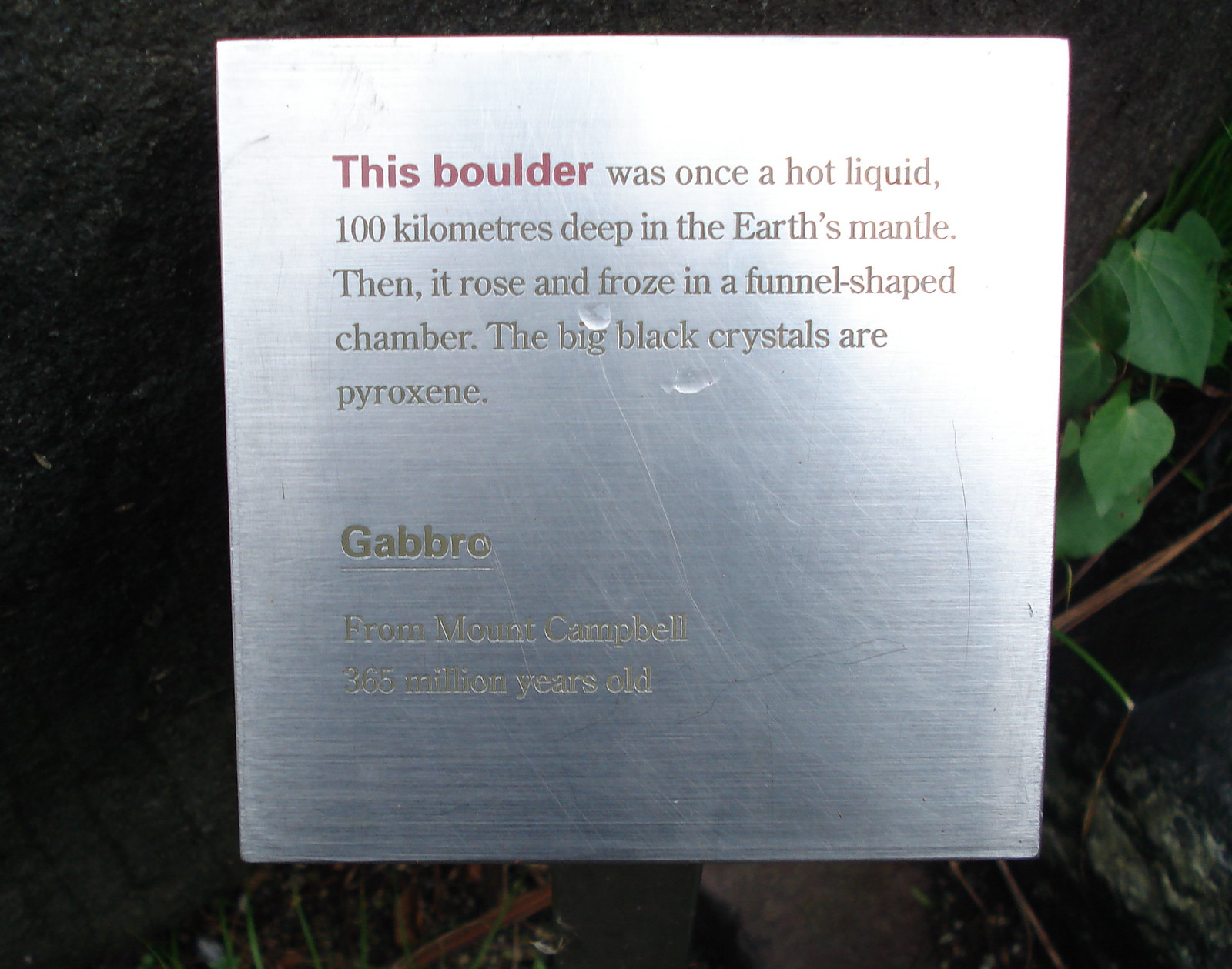The image depicts a metal sign with lightly etched gold text positioned outdoors or potentially within a museum setting. The sign's background is dark, but to its right, green leaves from a plant or bush are visible. The text on the sign includes the following details: in red, the initial phrase "This boulder," followed by light gray text that reads, "was once a hot liquid 100 kilometers deep in the Earth's mantle. Then it rose and froze in a funnel-shaped chamber. The big black crystals are pyroxene." Below this description, in smaller gold text, is the word "Gabbro," and further below, "from Mount Campbell, 365 million years old." The sign provides an informative background on the volcanic rock it accompanies, elaborating on its geological journey and composition.